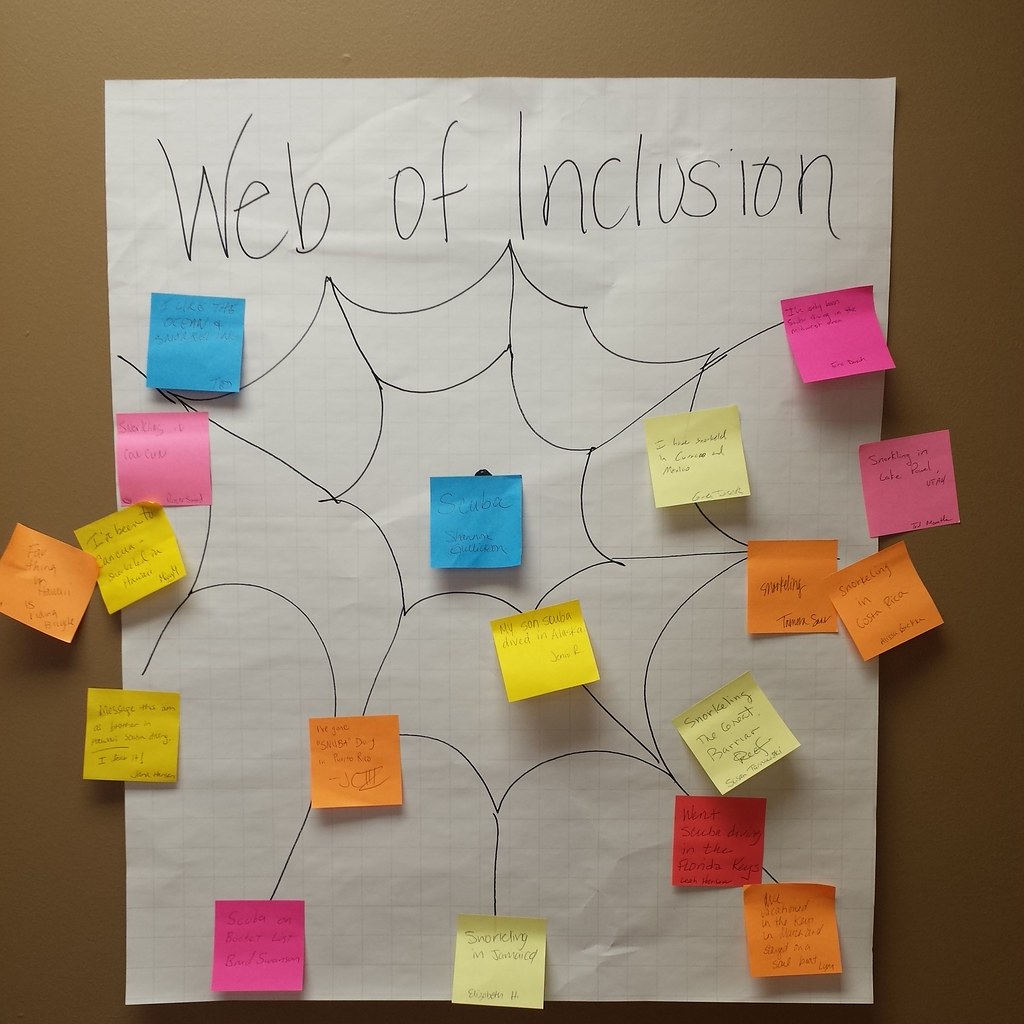This photograph features a homemade poster affixed to a brown wall. The large white sheet of paper bears the handwritten title "Web of Inclusion" at its top. A meticulously hand-drawn spider web, rendered in black ink, sprawls across the paper. Scattered throughout the web are 18 post-it notes in various vibrant colors, including turquoise, pink, dark pink, yellow, orange, red, blue, and purple. Each note contains some form of writing, though the text is too small to be legible in the image. The colorful post-its are randomly placed across different points of the web, creating a visually dynamic and inclusive mosaic of ideas or concepts connected by the web's tendrils.